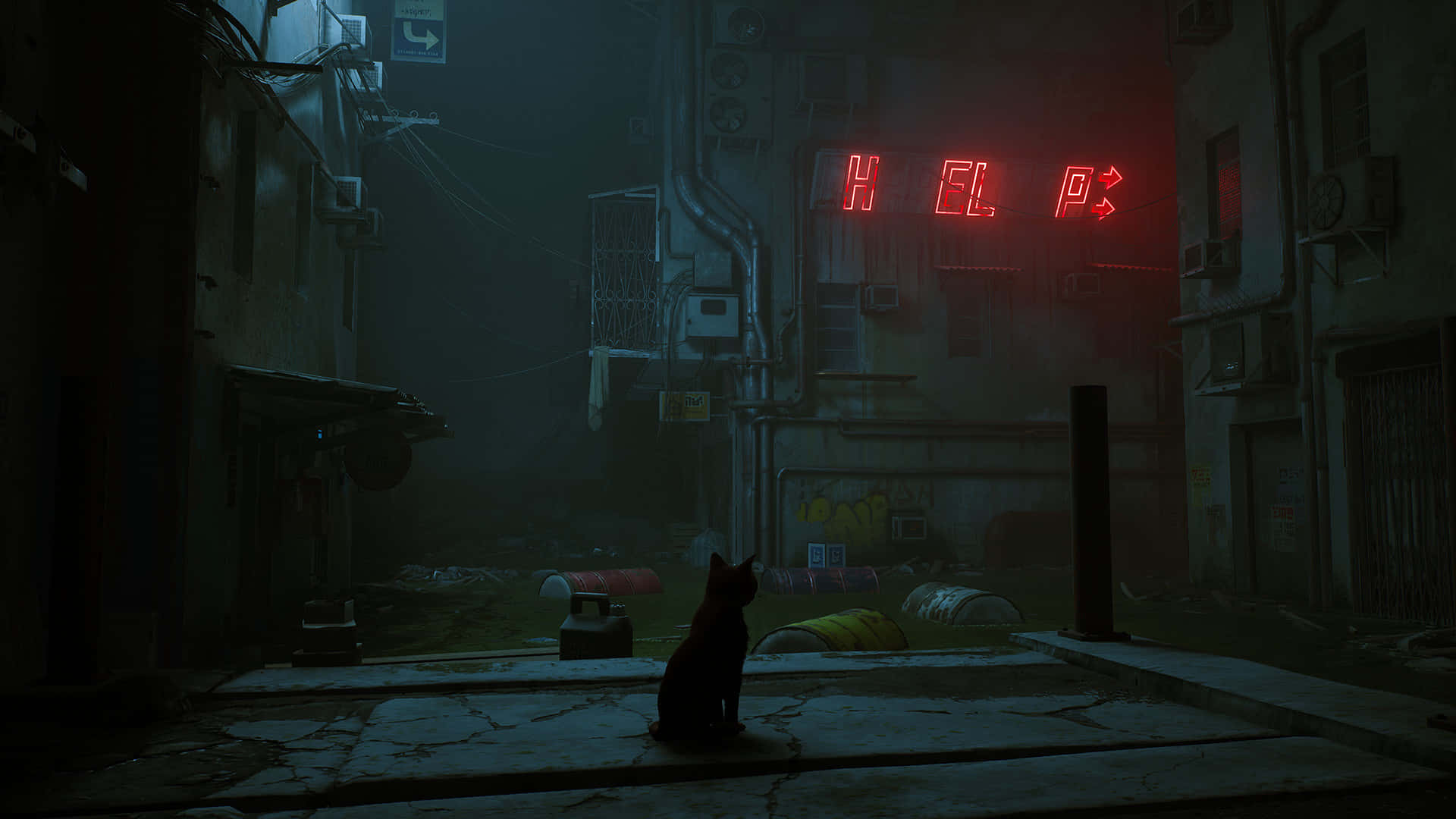In this detailed scene, which resembles a post-apocalyptic landscape straight out of a dystopian video game, the darkness of night envelops an abandoned, industrial setting. The image appears to be digitally crafted, though it’s unclear if it’s a photograph or computer-generated. A thin blue haze of light filters in from the top left corner, casting an eerie glow on the scene and illuminating a rectangular structure in the center. This structure is partially adorned with neon lights—most of which are malfunctioning—but the remaining illuminated red letters spell out the word "HELP", with two arrows pointing to the right. These letters stand out starkly against the dilapidated backdrop, suggesting the sign originally conveyed a different message. 

The scene is further characterized by a sense of neglect and decay: there are discarded steel drums of various colors, some floating in contaminated, flood-like waters that cover the streets. The setting evokes a sense of waste and pollution, contributing to the dire atmosphere. Along the edges of the buildings, tangled wiring hangs loosely, and one building features an elevated, screened-in porch, adding to the sense of disrepair.

In the foreground, the silhouette of a small, black cat sits on the sidewalk, staring upward at the ominous "HELP" sign. This detail adds an element of forlorn desolation, and the presence of mist and graffiti—scrawled on nearby walls—deepens the Blade Runner-esque aesthetic. Overall, the scene is marked by its dark, dank, and misty environment, with an unsettling, industrial ambiance that conveys a powerful sense of abandonment and urgency.